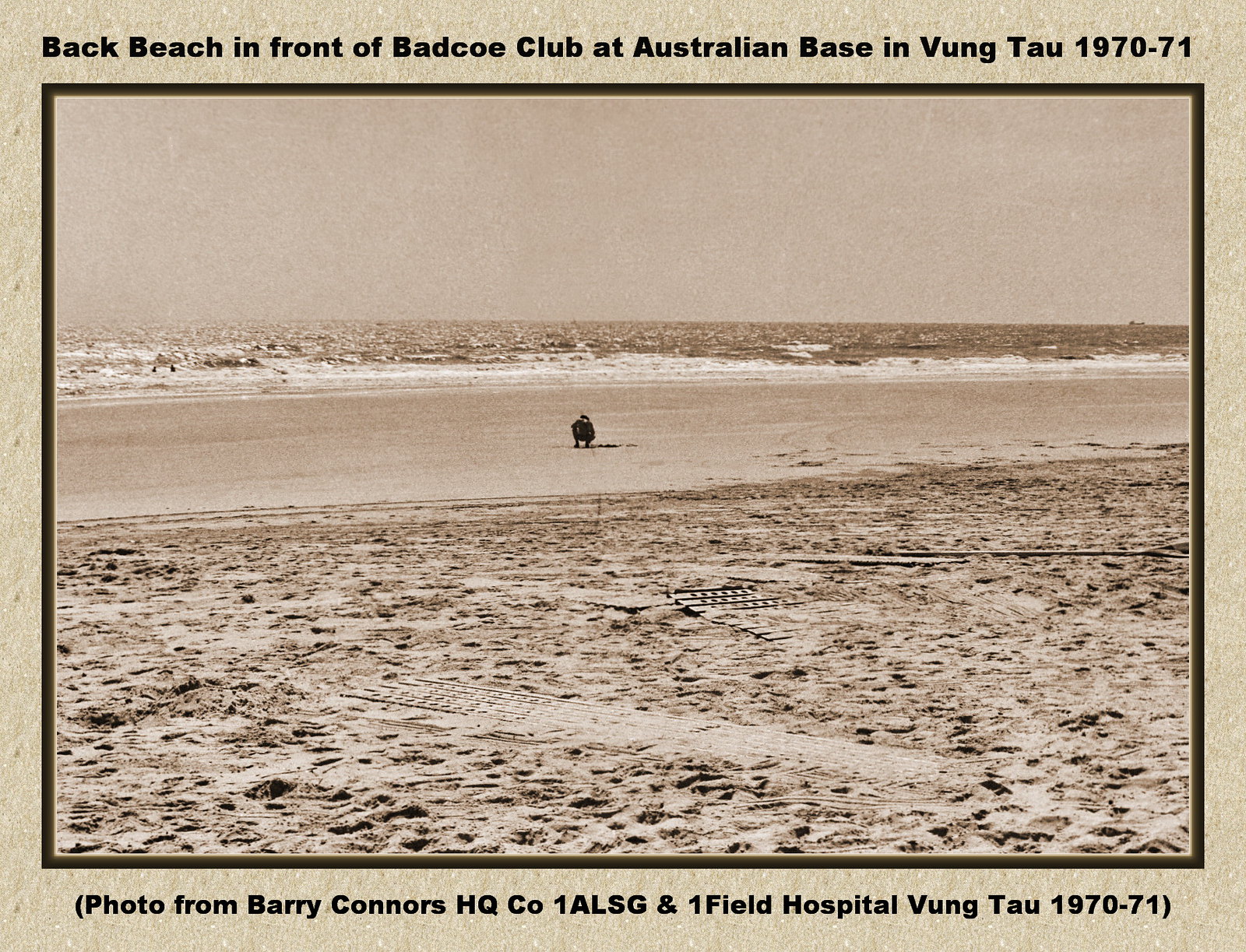This scanned postcard features a sepia-beige toned photograph taken at Back Beach in front of the BADCO Club at the Australian base in Vung Tau, during 1970-71. The text at the top of the postcard, in black, reads "Back Beach in front of BADCO club at Australian base in Vungtau, 1970-71." Below the main photograph, it notes, "Photo from Barry Connors HQ Co, 1 ALSG, & one field hospital, Vungtau, 1970-71." The photograph, bordered by black, captures a sunny day at low tide with gentle waves crashing on the beach. The sand in the foreground is marked by numerous footprints and tracks, possibly from vehicles. One person is seen crouching down, facing away from the camera, appearing to reach for something in the sand. There are other indistinct figures further out, possibly in the water. The background shows the beach extending into the distance, where the sand appears messy and wet, indicative of recent activity or debris. The image is superimposed on a white or tan colored cardstock, which shows individual fibers in the background, adding to the vintage feel of the scene.